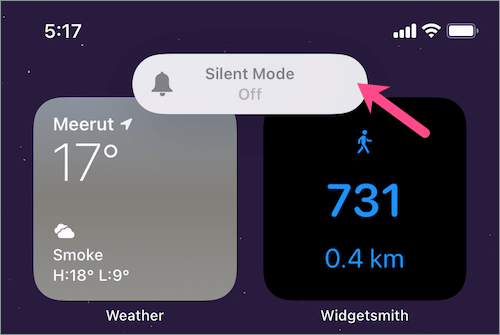The image displays a smartphone interface against a blue background. The device shows a detailed weather widget for Meerut, indicating a temperature of 17 degrees Celsius with an icon of clouds. The forecast shows a high (H) of 18 degrees and a low (L) of 9 degrees, accompanied by the label "weather." To the right, there is another square widget with a black background that features a blue 3D stick figure icon of a person walking, alongside the metrics "731" and "0.4 KM." At the bottom of this widget, the name "Smith" is displayed. The top of the image shows the time as 5:17 and the device is in silent mode, as indicated by a notification bell icon being highlighted with the label "silent mode off" within a light gray oval. Additionally, a red arrow points towards the light gray oval indicating "silent mode off."